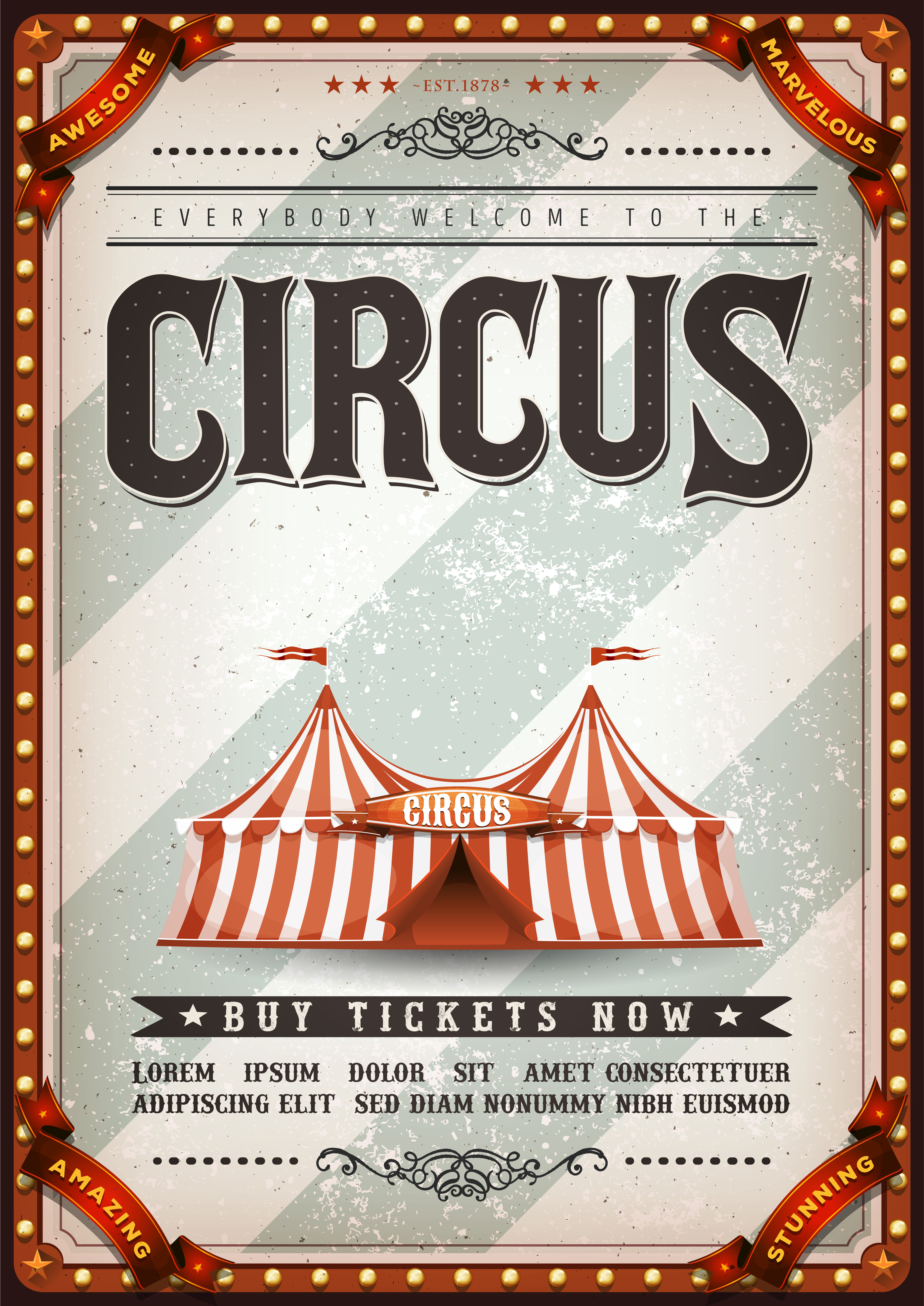This poster, designed in a vintage circus style, features a vertically aligned rectangular layout with an intricate border resembling marquee lights, complete with red borders adorned by gold dots. The background of the poster has diagonal stripes in varying shades of gray speckled with white spots. At the top, the poster displays three small red stars, followed by the text "EST 1878" flanked by three more red stars. 

Beneath this, the text reads "Everybody Welcome to the" in dark lettering, leading to the word "Circus" prominently displayed in large dark block letters with white outlines and tiny gray dots running through them. Below this, the visual centerpiece is an image of a red and white striped circus tent with two triangular peaks, each topped with a small flag flying in opposite directions. The tent dips in the center, where "Circus" is written in white letters.

Further down, a small star precedes a black banner with bold white text that says "Buy Tickets Now," followed by another star against a dark brown background. The bottom section includes placeholder Latin text, most likely used for design purposes, reading "Lorem Ipsum Dola Sit Amet Consectactua Adispinsim Elisidiam Nomnummi Nibh Euismod."

In the left and right corners, red banners proclaim the words "Awesome," "Marvelous," "Amazing," and "Stunning" in vibrant red letters, enhancing the eye-catching allure of this classic circus advertisement.